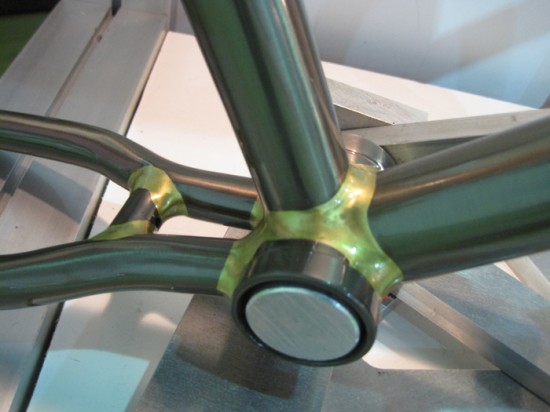The photograph features a close-up of an intricate metal structure that resembles the central portion of a bicycle frame, with an array of shiny, glossy greenish-black rods or pipes welded together. These metallic pieces converge in the center where they are connected by gold-colored clasps and a black cylindrical protrusion topped with a silver disc. The background is largely white, possibly a wooden board, accented with patches of blue light on the bottom left and pinkish-orange light on the top left. Additionally, a grey painted wood slab is visible on the left side of the photo, adding to the composition.